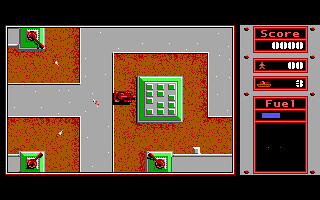This image appears to be a screen capture from a video game, showcasing an intense battle scenario. On the right side of the screen, there is a vertical rectangular info panel. At the top of this panel, the player's score is displayed, showing zero points. Just below the score, two remaining lives are indicated. Further down, another box reveals that the player has three tanks available, with an accompanying icon depicting a military tank. Below this, a large black box features a blue fuel bar that is halfway depleted, indicating the player has around 50% fuel left.

On the left side of the image, a single tank is aimed at a green building, which is situated on sandy-colored soil. Additionally, the screen shows three enemy guns targeting the red tank: one on the top left, another on the bottom left, and the third near the middle bottom of the picture. The visual composition suggests a strategic and potentially hazardous situation for the player in this virtual environment.